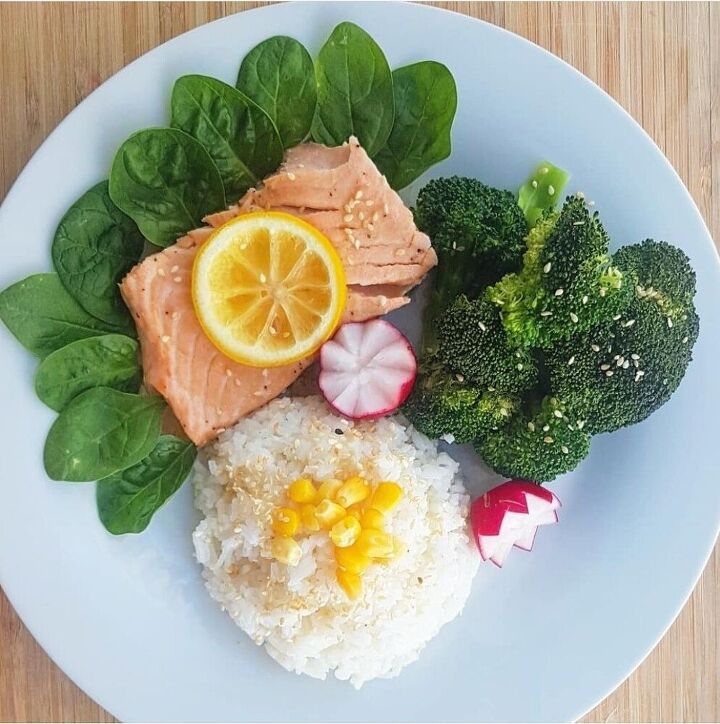The image shows a close-up of a round, pale blue pottery plate, which is sitting on a light wooden tabletop. The plate features a decorative and appetizing arrangement of food. In the upper left section, baby spinach leaves are neatly placed, creating a bed for a fillet of pink salmon, garnished with a slice of lemon on top. The salmon itself is also sprinkled with sesame seeds. Adjacent to the salmon on the right side of the plate are broccoli florets, similarly topped with sesame seeds. Towards the bottom of the plate, there is a scoop of white rice adorned with a few pieces of corn kernels. Adding an extra touch of elegance, radishes, cut into flower shapes, are placed thoughtfully as garnish.